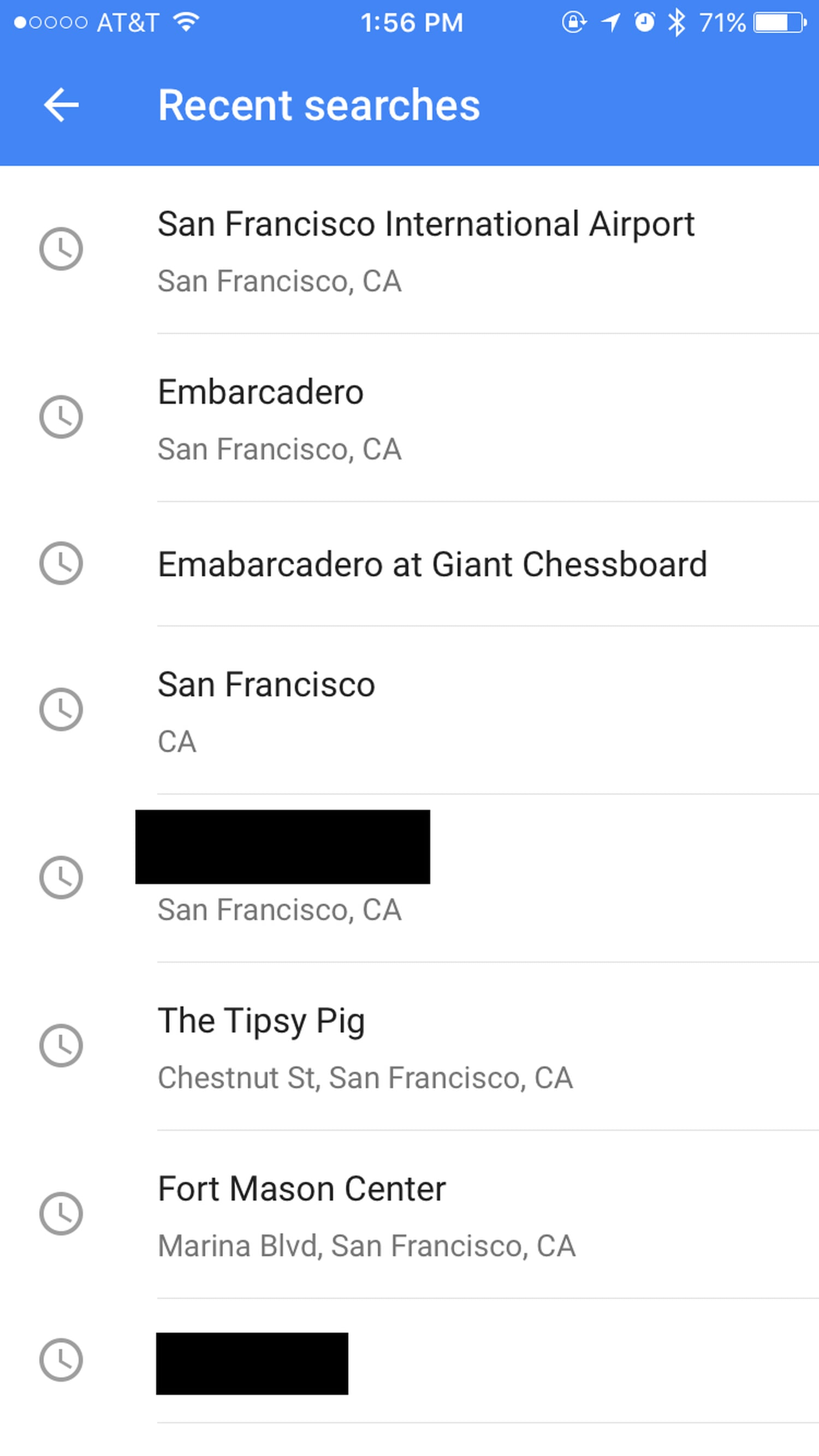A screenshot of a phone display shows the recent search page from an AT&T mobile device. The time displayed is 1:50 PM and the battery is at 71 percent. The top part of the screen features a blue stripe with all text in white, including "Recent Searches." Below the blue stripe, the background is white with black text listing several recent searches. These searches include: 

1. San Francisco International Airport, San Francisco, California
2. Embarcadero, San Francisco, California
3. Embarcadero, a giant chess board
4. San Francisco, California
5. [Redacted entry]
6. The Tipsy Pig, Chestnut Street, San Francisco, California
7. Fort Mason Center, Marina Boulevard, San Francisco, California
8. [Another redacted entry]